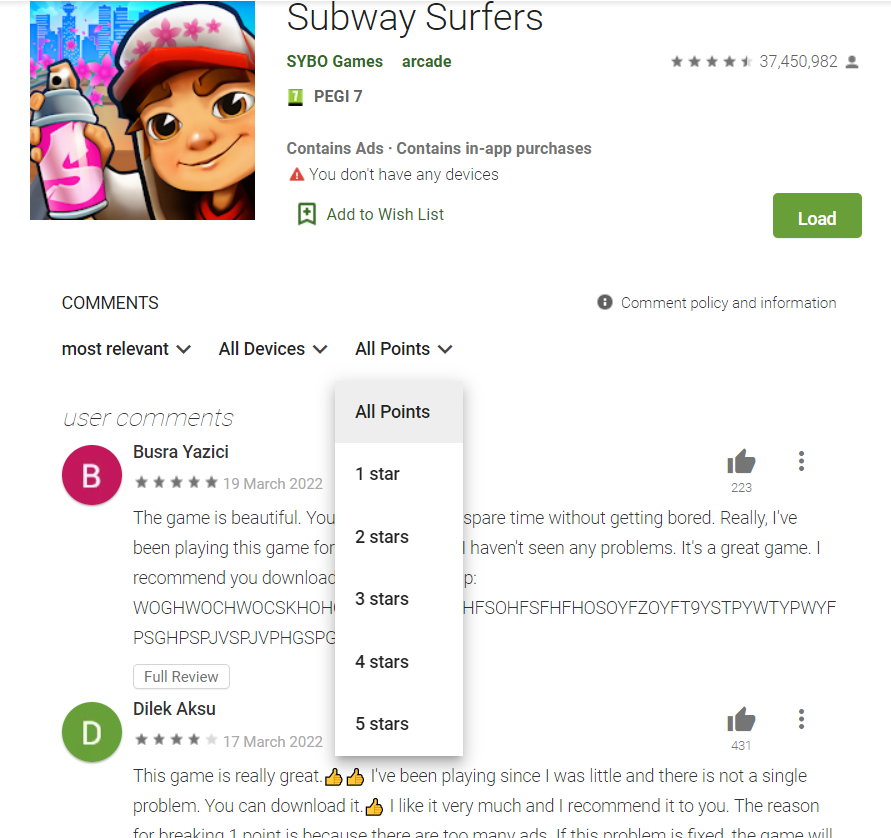The image displays a website page featuring the game "Subway Surfers" by SYBO Games. At the top of the page, there is a square graphic showcasing a cartoon figure of a girl standing against a cityscape backdrop. The girl is holding a spray paint can and is styled with a baseball cap, thick brown eyebrows, brown eyes, and long brown hair. Adjacent to her image, the text "Subway Surfers" is prominently displayed. Below this, the information "SYBO Games, Arcade, Contains ads, Contains in-app purchases" is provided.

Further down the page, a comment section is visible. It features options such as "Comments," "Most relevant," "All devices," and "All points." The "All points" filter is selected, with a drop-down menu showing rating options from one to five stars. Below this, user reviews are displayed, beginning with the latest comments.

The first review is by a user named Bursa Busra Yazici, represented by a dark magenta circle with a capital 'B' inside it. Bursa’s review is fully visible. The second review is by a user named Dilek Aksu, denoted by a green circle with a white capital 'D.' However, their review is partially cut off, making the entire content unreadable.